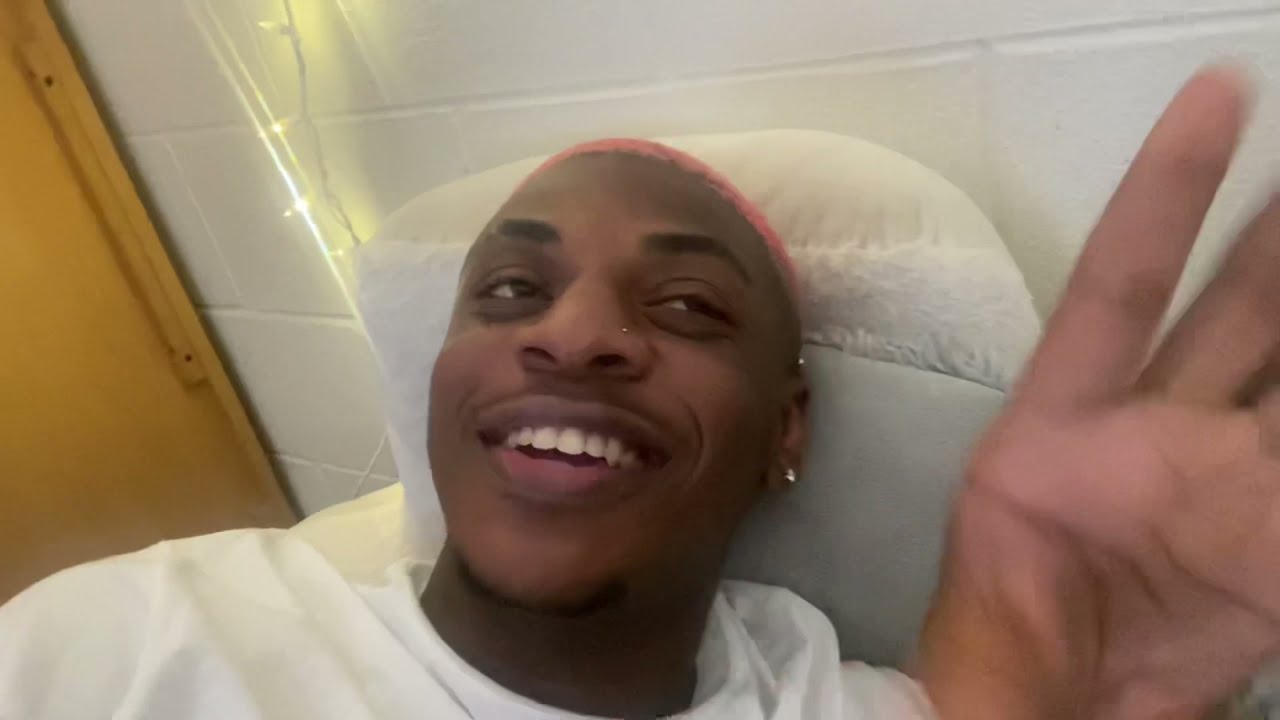In the image, a young black man is laying his head on a white pillow against a white cinder block wall, possibly in a dorm-like setting. His bright, very short pink hair contrasts with his white plain t-shirt, and a small silver stud earring can be seen in his left ear. He has a slight facial hair on his chin. The man is smiling warmly, looking slightly up and to the left, engaging with someone or something outside the frame. His left hand is lifted with the palm facing upward. The background features softly glowing white Christmas lights and to the left side of the picture, a yellow wall and a tall cabinet or armoire are partially visible. This scene evokes a candid and intimate moment, possibly captured during a video call.